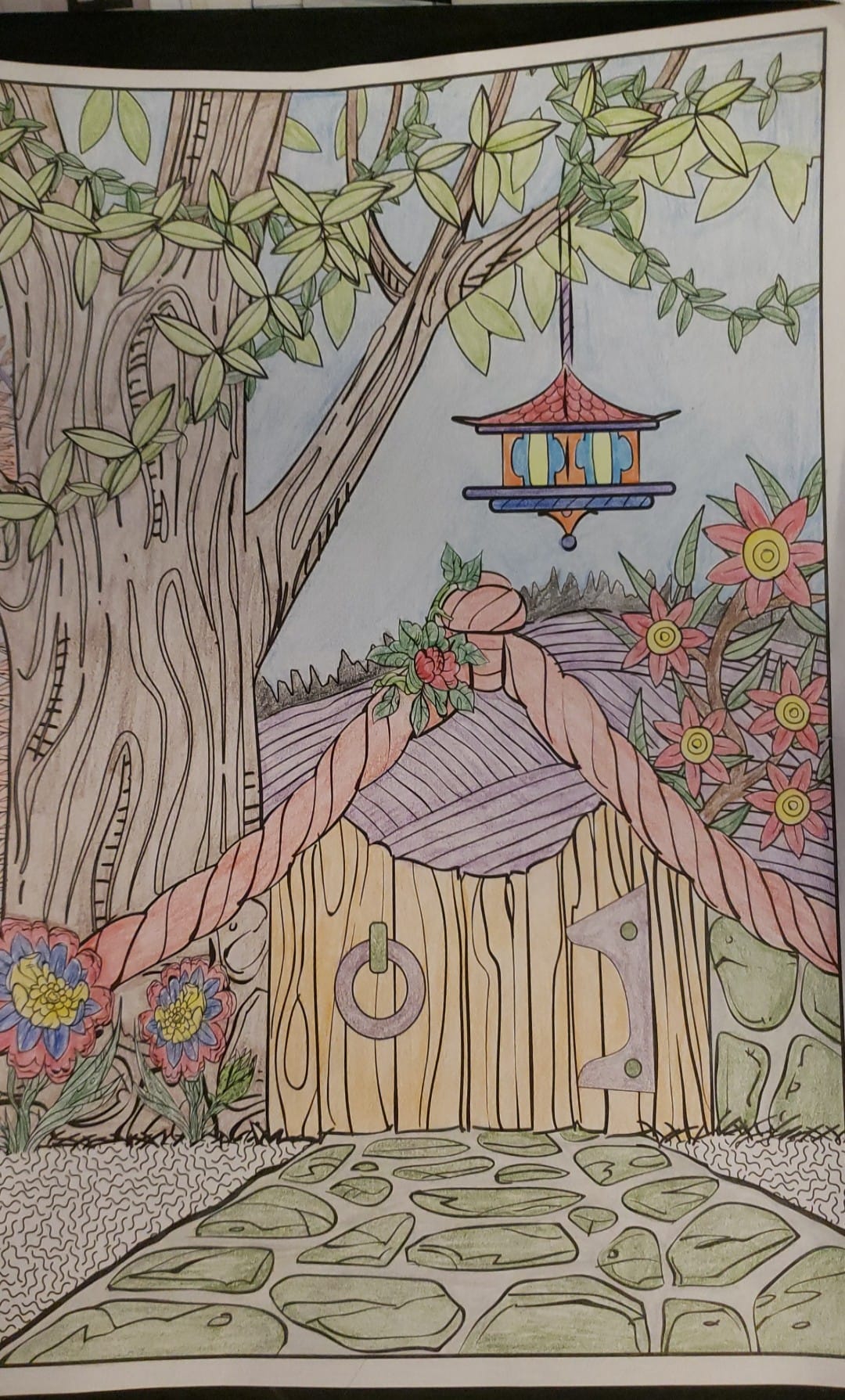An illustration with a black background showcases a charming, cartoonish scene drawn on a light purple piece of paper. The focal point is a whimsical tree with light brown bark and lush green leaves. Hanging from a thin rope on the tree is a colorful birdhouse. The birdhouse features a red roof that curves upward at the ends, decorated with accents of yellow, blue, and red along the edges. Its bottom is painted purple, and it has a pointed red finial.

In the background, thick ropes are tied off over a wooden fence, which is partially open and revealed by a large, round iron gate latch. The scene is adorned with vibrant pink and yellow flowers scattered among gently rolling hills and patches of greenery. A stone pathway winds through the foreground, flanked by neatly trimmed grass on either side.